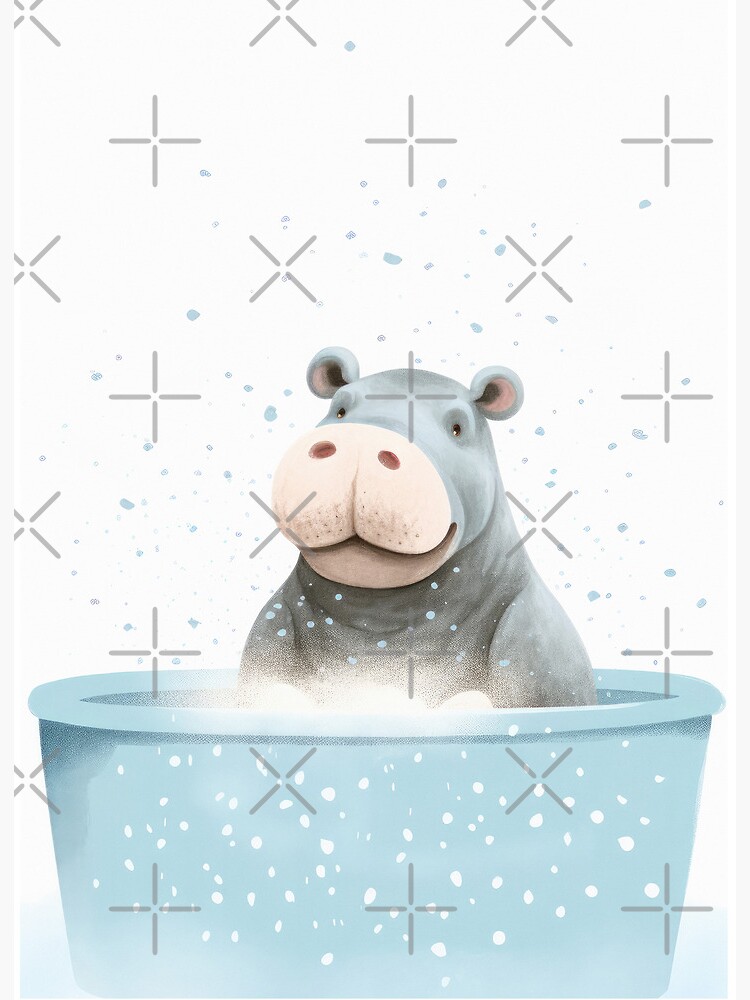This image is a playful, digital illustration ideal for a child’s bathroom or bedroom. It features a happy hippopotamus sitting in a circular, cyan-colored bathtub. The hippo, which has a dark gray skin with splashes of light gray, is positioned slightly below the center of the white background with its chest and head visible. The hippo’s large pink snout, small black eyes, and circular ears with pink interiors contribute to its endearing appearance. The bathtub is producing small waves of white foam due to the hippo's movements, and there are water droplets around it, adding to the lively atmosphere. Surrounding the image are alternating rows of transparent gray crosses and X's, designed to prevent unauthorized copying. The overall muted tones of gray, blue, and pink give the illustration a soft, stuffed-animal-like quality, making it perfect for hanging in a nursery or young child's space.